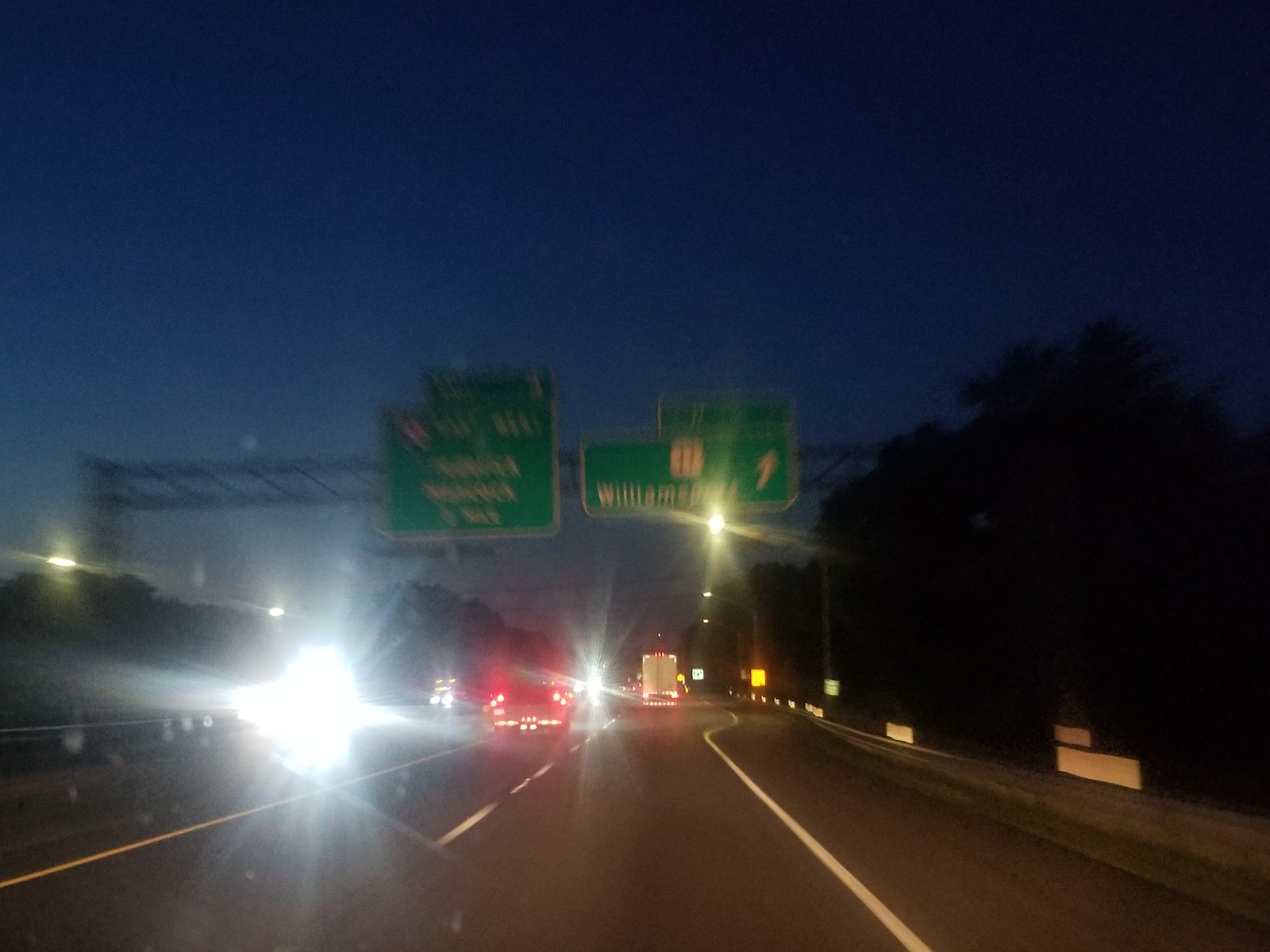This night-time dash cam image, likely captured from a camera affixed to a car's hood, presents a highway scene in motion. The dark blue sky hints at twilight hours, though the absence of the car's hood suggests the camera's position may be on the external front of the vehicle. Blurriness adds a sense of motion, as the lanes and trees, shrouded in darkness, streak past. The trees, laden with leaves, blend into the night, appearing almost black. Two large, green highway signs mounted on a metal post span the image. Despite the blur, one sign, rectangular and more distinct, reads "Williamsport," while the other, more squared sign, remains illegible. This photograph encapsulates the fleeting scenery typical of a late drive on a bustling highway.